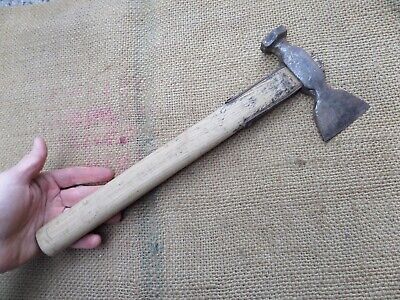The image showcases a close-up of a multi-functional tool resting diagonally at a 45-degree angle against a rough, textured burlap background. The tool features a light beige, thick wooden handle, which appears dirty and scratched near the top, with blackened, stained metal components. One end of the tool serves as a hammerhead while the opposite end functions as an axe or flat blade, suggesting its versatility for both pounding and scraping tasks. A man's left hand enters the frame from the left side, palm facing upwards, with the thumb extended. The hand, appearing pale, either has just placed the tool down or is in the process of picking it up, with the handle laying across the palm and wrist. The image captures a moment poised between action and rest, highlighting the blend of utility and wear in the tool's design.